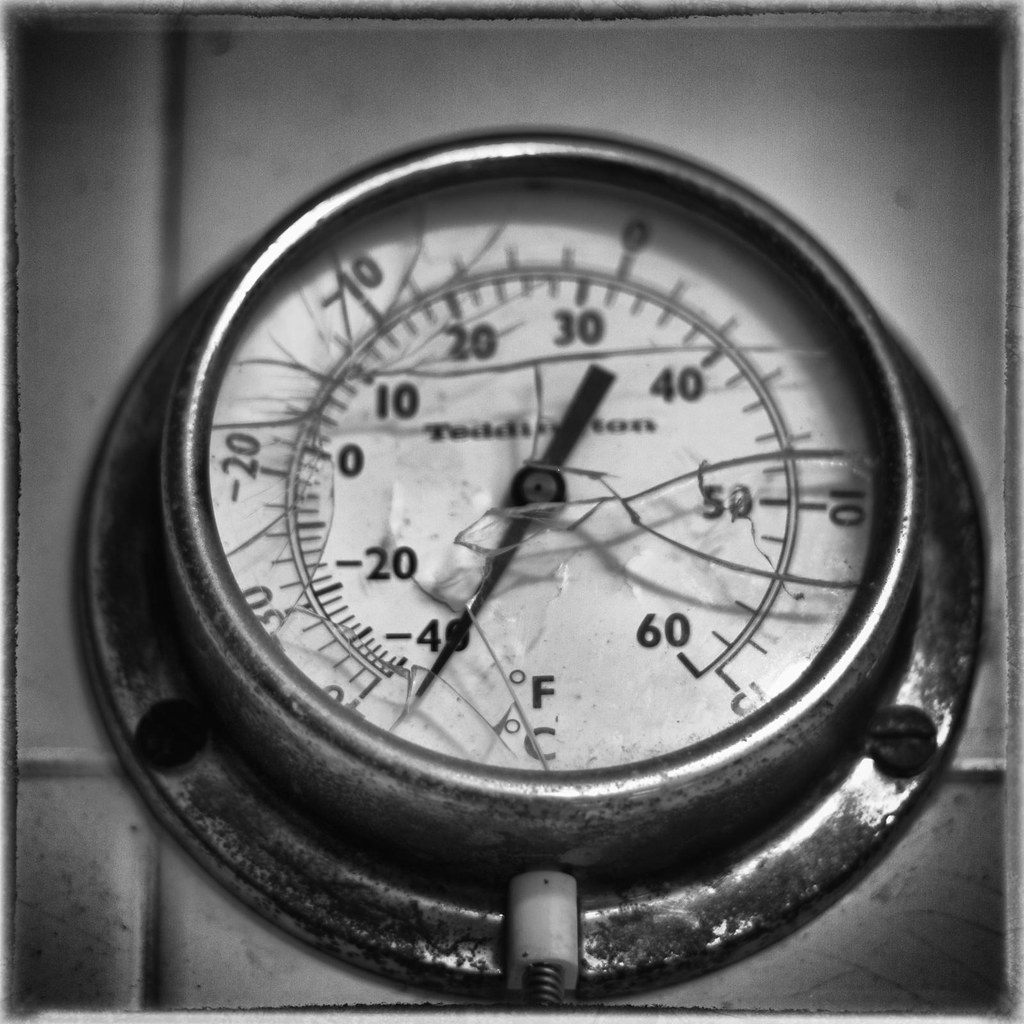The black and white photograph depicts a thermometer with a metallic base, set on a tiled surface. The center of the device prominently features a dial that displays temperature readings in both Fahrenheit and Celsius. The temperature gauge ranges from -40°F to 60°F in a circular arrangement, with corresponding Celsius values. The glass covering the meter is visibly cracked, adding a vintage or worn appearance to the instrument. Although the brand name of the thermometer is positioned at the center of the dial, it is partially obscured and difficult to read, appearing to be something similar to "TEDDON" or a variation thereof. The thermometer's indicator needle points to the -40°F mark, suggesting either it is turned off or denotes an extremely low temperature reading.